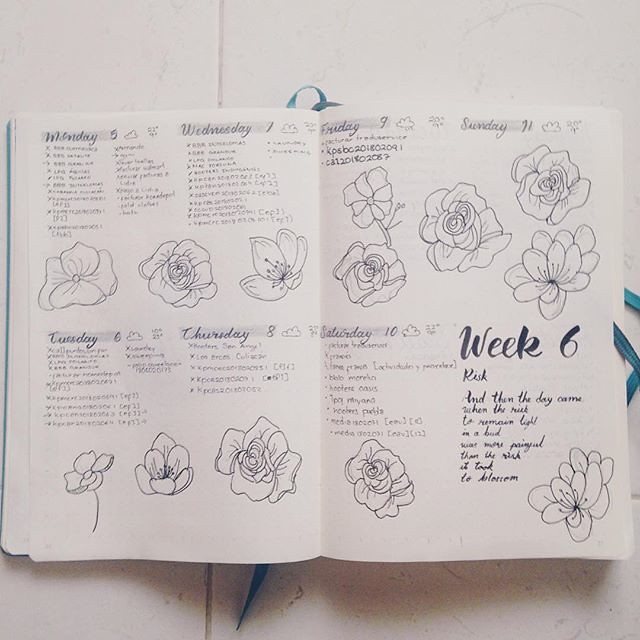This image captures an open book laid out on a white, tiled surface, clearly showing its white pages filled with delicate black-ink drawings of flowers. Each day of the week is methodically listed across both pages: Monday, Wednesday, Tuesday, Thursday on the left, and Friday, Sunday, Saturday on the right. The focus is on a segment marked "week six," prominently displayed in bold black script, with the word "risk" beneath it, followed by a nearly illegible poem. Each day is accompanied by what appears to be small, handwritten checklists, difficult to decipher, suggesting a structured journal or diary, possibly with a floral theme. Blue ribbon bookmarks are subtly visible in the background, adding a touch of color against the minimalist white setting.